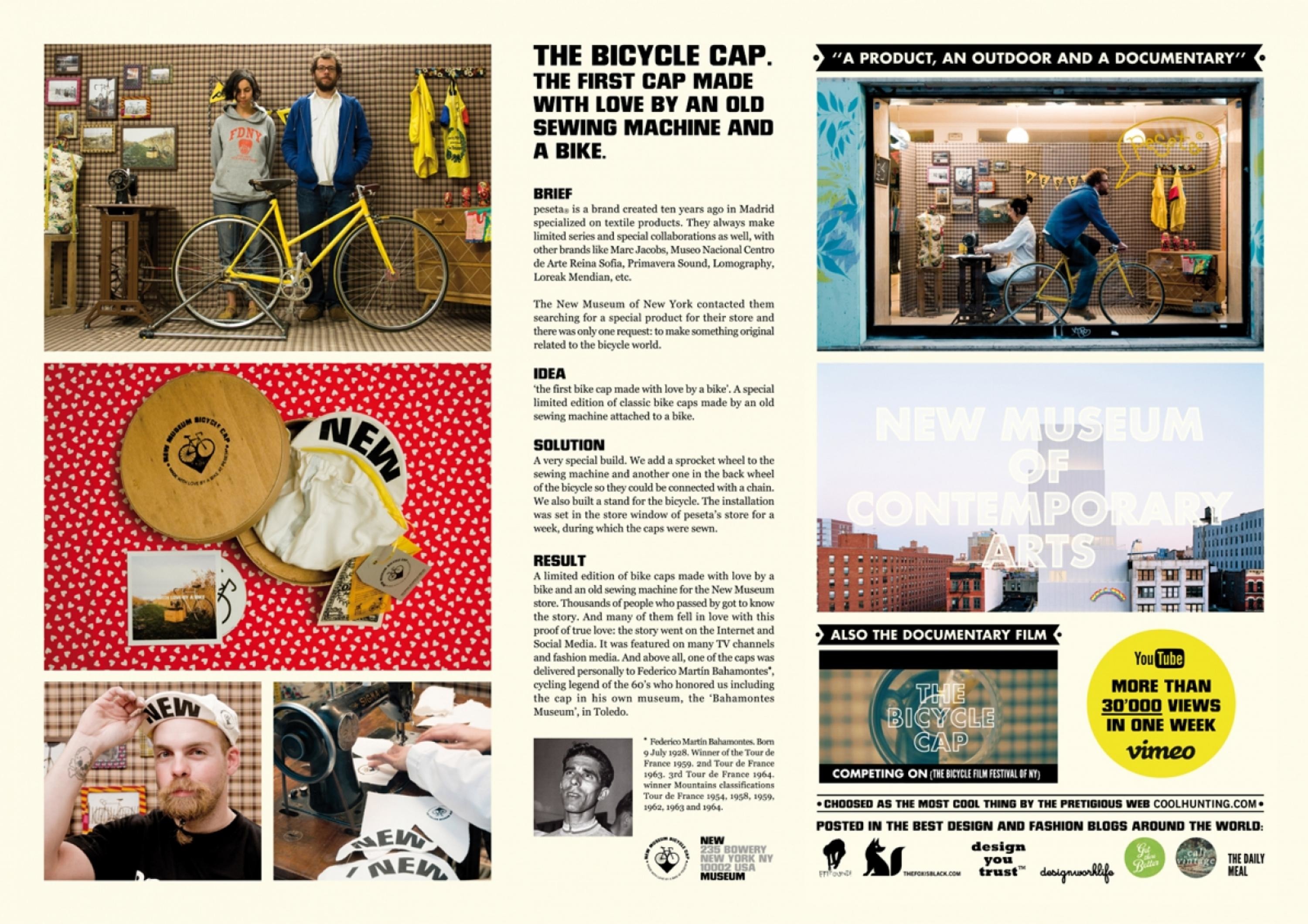This advertisement for the Museum of Contemporary Art in New York is presented on an off-white background and is divided into three vertical columns. The central column features a detailed, text-based narrative about the history of the bicycle cap, broken into sections titled "Idea," "Solution," and "Final Result," and includes a small black-and-white photograph of the author. The side columns (first and third) showcase a series of images. 

On the left, the first column begins with a photograph of a man and a woman standing in front of a yellow bicycle inside what appears to be their shop, adorned with pictures and shirts. This is followed by a picture with a red tabletop adorned with white hearts displaying the bicycle cap alongside assorted Polaroid photos in an artsy layout. Two smaller photos show a man wearing the cap and another individual working on a sewing machine – implied to have crafted the first bicycle cap with love.

The third column, labeled "Product, Outdoor, and Documentary," starts with an image of people standing behind a building window, mimicking mannequins. Below that is a skyline photograph with the words "New Museum of Contemporary Art" superimposed. The rest of the column contains smaller, intricate images, including a YouTube icon, various logos, and company names that become challenging to discern.

Overall, the advertisement effectively combines visuals of bicycle caps and their creators, with a rich narrative history, showcasing the exhibit at the museum.